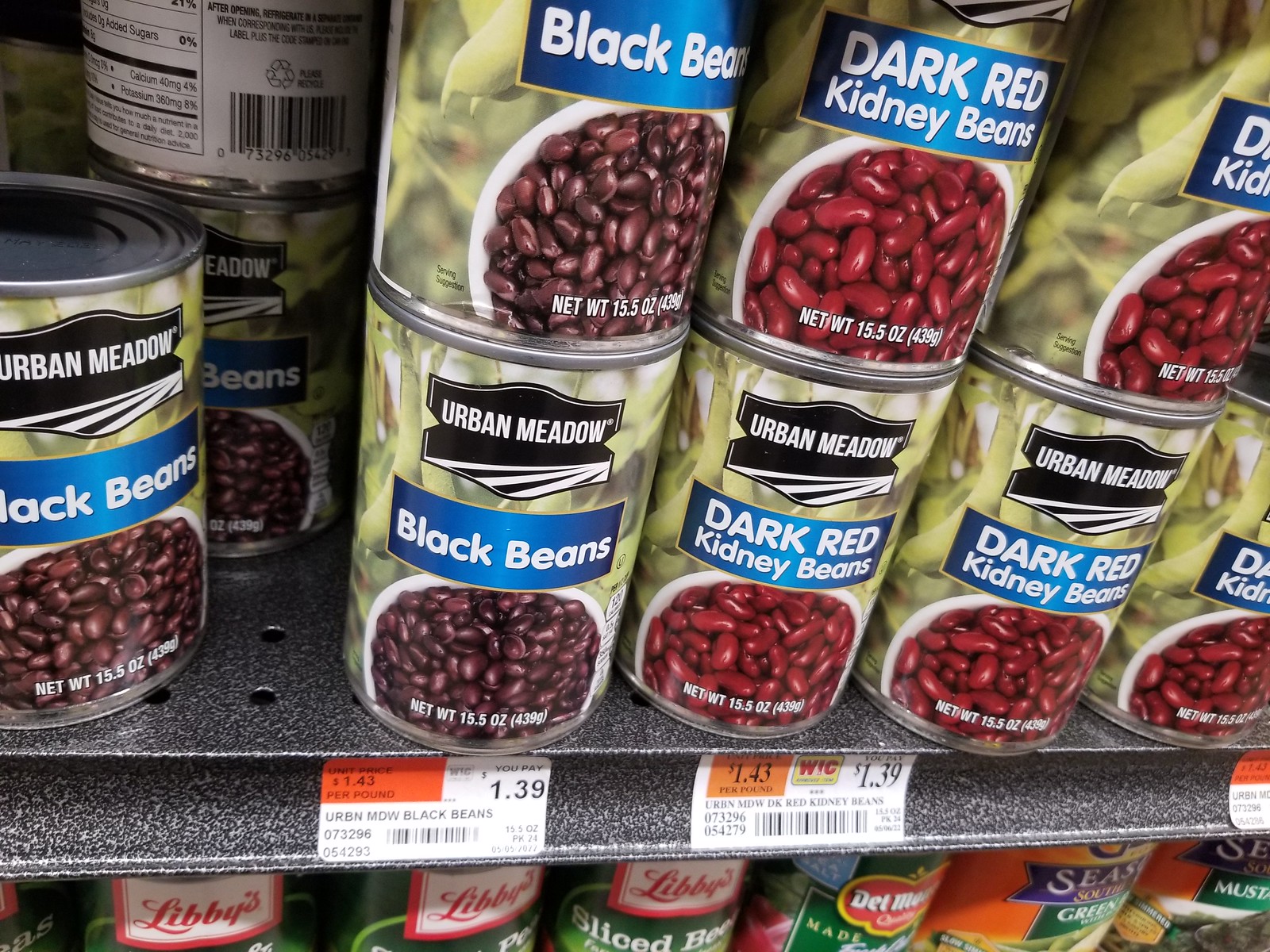The image depicts a well-organized grocery store aisle with neatly shelved products. Prominently displayed are rows of canned goods, specifically featuring black beans and dark red kidney beans from the brand Urban Meadow. These Urban Meadow cans feature a black and white logo centered on their blue labels, accompanied by black font and a bean illustration. Price tags are visible beneath these cans, indicating the cost of the products.

On the shelf below, more canned goods are arranged, including selections from the brand Libby's, although the specific types of Libby's products are indistinct. Additionally, there are cans from Del Monte, which appear to contain a green, seasoned product. Overall, the store aisle is well-stocked and meticulously organized, providing shoppers with a variety of canned food options.